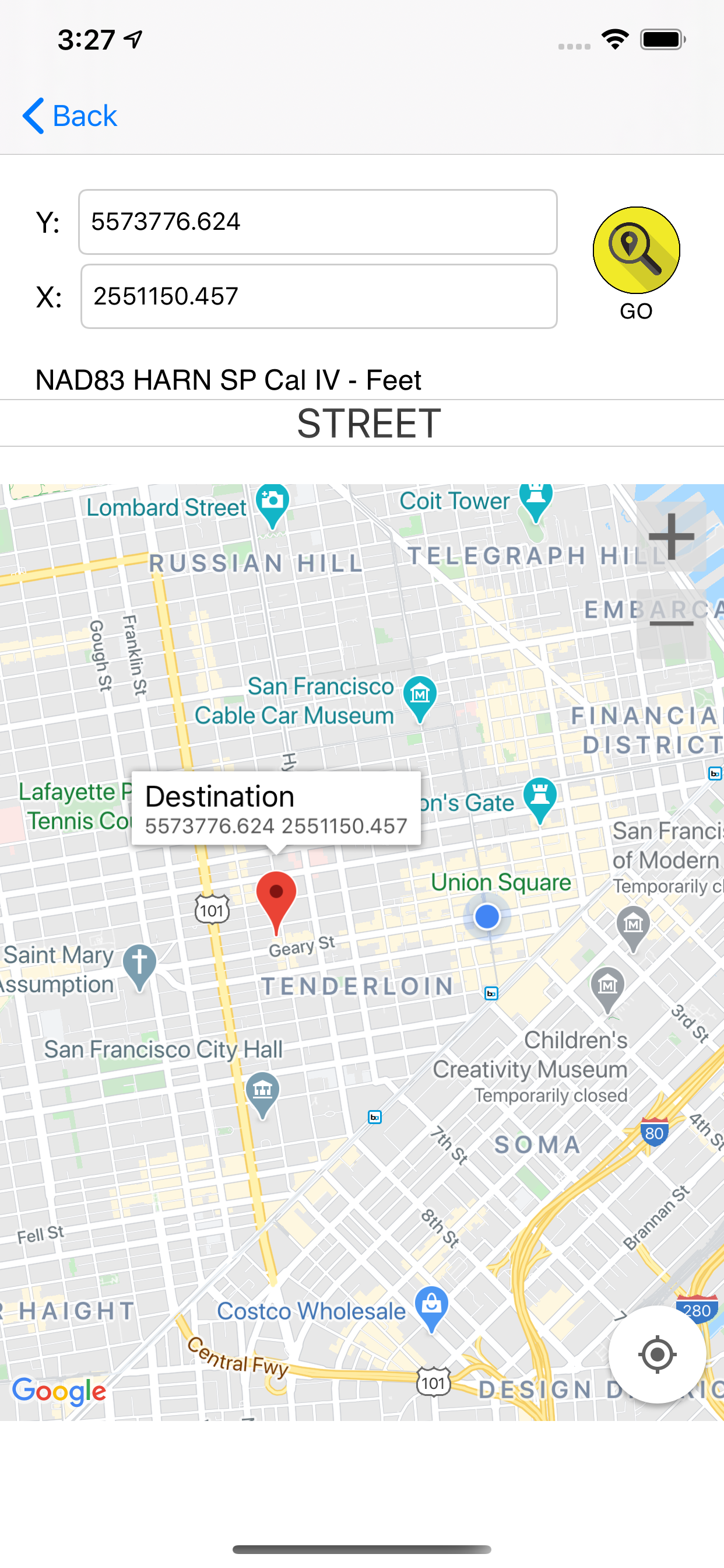This is a vertical screenshot from a mobile device, likely an iPhone or Android. At the very top of the screen, a gray status bar displays the time "3:27" in the upper left-hand corner, accompanied by a black triangle icon pointing to the upper right. Adjacent to the right, there are four gray dots, followed by a black Wi-Fi symbol, and a full battery icon.

Below the time, there's a blue, sideways 'V' icon with the label "Back" beneath it. Immediately under this, there is a white rectangular section containing two lines of text. The first line reads "Y: 5573776.624," and the second line reads "X: 2551150.457," which appear to be coordinates. To the right of these coordinates is a yellow circle featuring a black magnifying glass with a black location pin in its center. Beneath the coordinates, large black letters spell out "NAD83 HARN SP CAL IV-feet," flanked by two thin gray lines.

This section is followed by the word "Street" in bold black letters. Below this, there is a square map displaying a portion of downtown San Francisco. Recognizable areas such as the Tenderloin, Russian Hill, and Telegraph Hill are labeled in gray on the map. White streets intersect with larger yellow roadways, including US 101 and Interstate 80, indicated by highway shields.

In the upper left corner of the map, a white box with black text reads "Destination," and underneath it, the coordinates from above are replicated. To the right, two gray boxes stacked atop each other contain plus and minus signs for zooming in and out. In the bottom right corner of the map, there is a white circle with a gray icon, possibly a centering button.

Finally, at the very bottom of the screen, a long thin gray bar extends across the width of the screenshot.